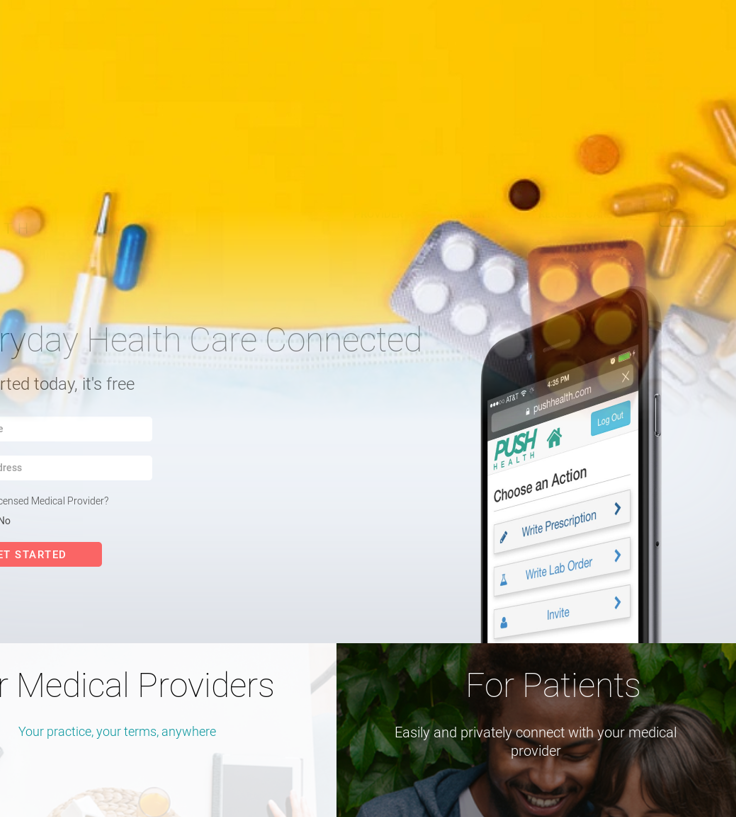This image appears to be a partial screenshot of a healthcare-focused website's homepage, capturing primarily the right half of the layout. The top third of the image features a yellow background, which transitions into white, evocative of a mask, blending overlaid images of various pills.

Text on the page is partly obscured. The phrase "every day healthcare connected" is visible with the first part of "every day" cut off, leaving only "R-Y-D-A-Y." Below this, it seems to start with the fragmented "R-T-E-D" and continues "started today, it's free." 

Two input fields are positioned beneath this text, accompanied by links to licensed medical providers and another truncated link. A prominent red button labeled "Get Started" in white font is centered below these elements.

To the right, an illustration of a smartphone displays the website, identified as "pushhealth.com." The phone screen shows options such as writing a prescription, placing a lab order, or sending an invitation.

Towards the bottom, two boxes are present. The left box, with a white background and cutting off part of the text ending in "R," states "Your practice, your terms, anywhere" in blue font. The right box features two smiling individuals facing downward, surrounded by vibrant green leaves, with content partially cut off.

This partial glimpse into the website suggests a modern, digital healthcare service aimed at making medical services more accessible and interconnected.